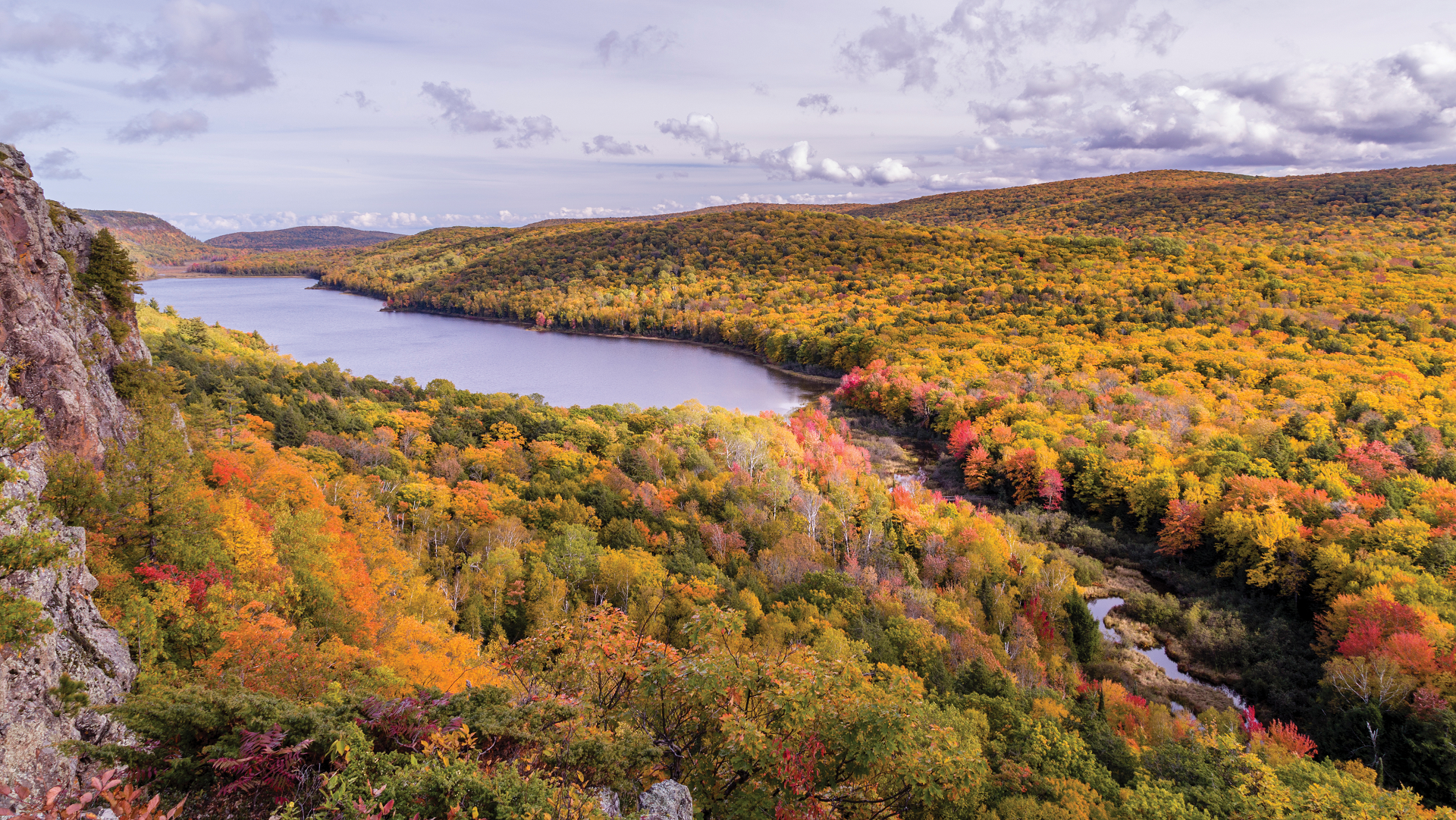The image depicts an aerial view of a lush, expansive forest in the midst of autumn, with a vibrant mix of orange, red, yellow, green, and russet-colored foliage. A winding river, starting as a small lake, cuts diagonally through a green valley covered in various types of trees and flows toward the top left of the image. On the left side, a rocky crag or the side of a mountain adds a rugged touch to the scene, while rolling hills can be seen in the far distance. The sky above is mostly clear, adorned with gray, puffy clouds, casting a serene atmosphere over the wilderness setting.